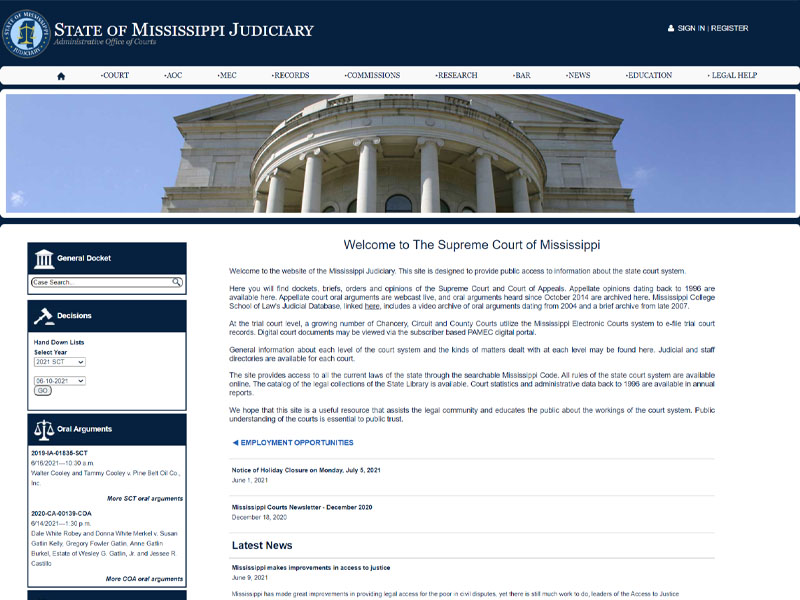The image features a structured layout designed for the State of Mississippi Judiciary's webpage. At the top of the image is a blue border with the text "State of Mississippi Judiciary" prominently displayed. Directly below, there is a white section with several clickable areas labeled "Court," "Commission," "Education," and additional labels that are too small and blurry to discern.

Beneath this, the image showcases a photograph set against a blue sky background. The photo captures a grand building, with a dome supported by marble columns. Below the image, the text "Welcome to the Supreme Court of Mississippi" is clearly visible.

The lower portion of the image contains several paragraphs of text that are too small and blurry to read. Further down, there are light gray horizontal lines with accompanying text above each line, also too small and blurry to decipher.

On the left side, there is a vertical menu. The top of this menu features text that is similarly too small and blurry to read. Beneath this menu, there is a text box where users can type in information. At the bottom, there is a blue section featuring the image of a gavel.